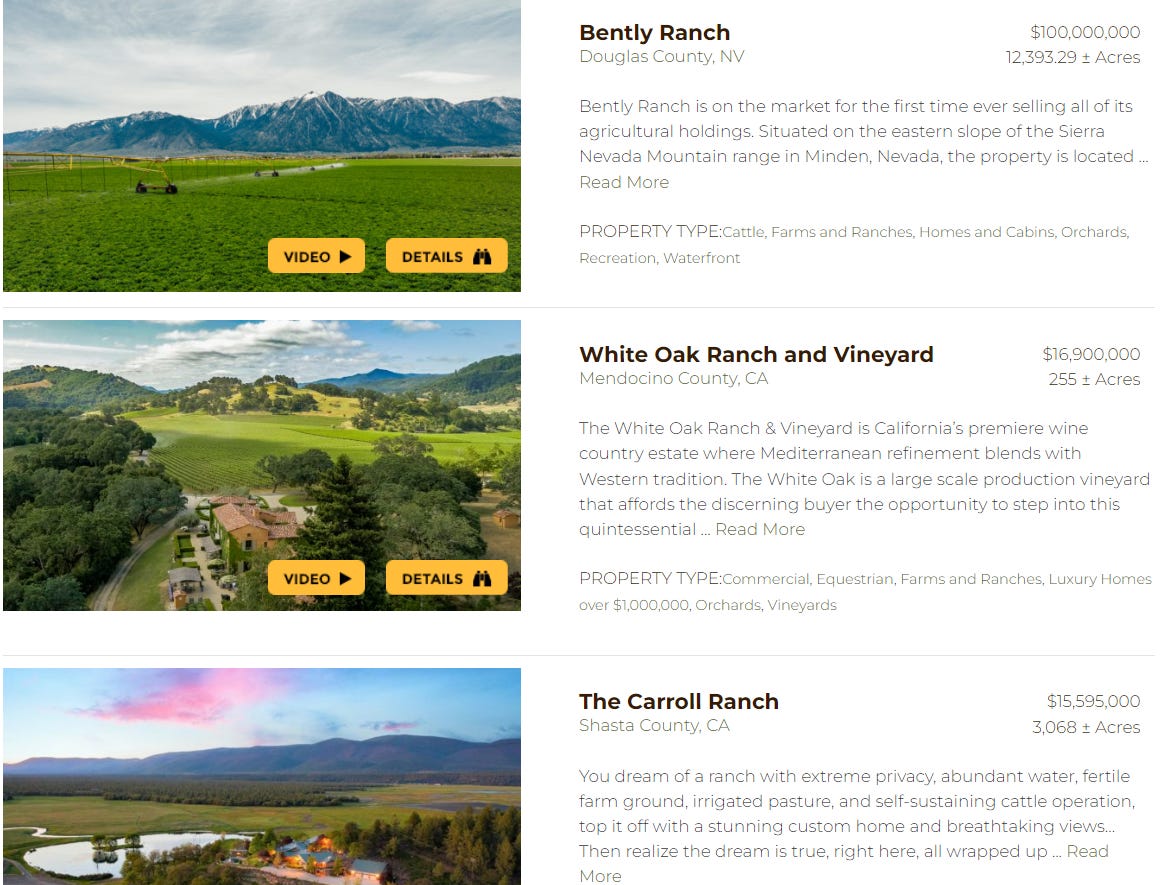The image showcases a collage comprising six smaller pictures arranged in two columns. On the left, there are three pictures displayed vertically, while the three on the right side appear to be explanations matching the images on the left. 

At the top, the first picture captures an expansive, open grassy area. The foreground is dominated by verdant fields, giving way to a majestic backdrop featuring a mountainous view. The peaks are partially snow-capped, suggesting a high elevation. Above, the sky is slightly overcast with wispy, white clouds dispersed throughout, creating a serene and picturesque landscape. Towards the bottom of this picture, there is a yellow rectangular label with black text that reads "Video" and "Details".

Adjacent to this image, the corresponding explanatory text details the location as Bentley Ranch in Douglas County, Nevada. The description indicates that this property, encompassing valuable agricultural holdings on the eastern slope of the Sierra Nevada mountain range, is on the market for the first time ever. The asking price is prominently stated as $100 million, along with the cost per acre.

Below this, the description shifts focus to two other properties mentioned: White Oak Ranch and Vineyard, followed by Carroll Ranch in California, implying that these are possibly other listings or features detailed within the same exposition.